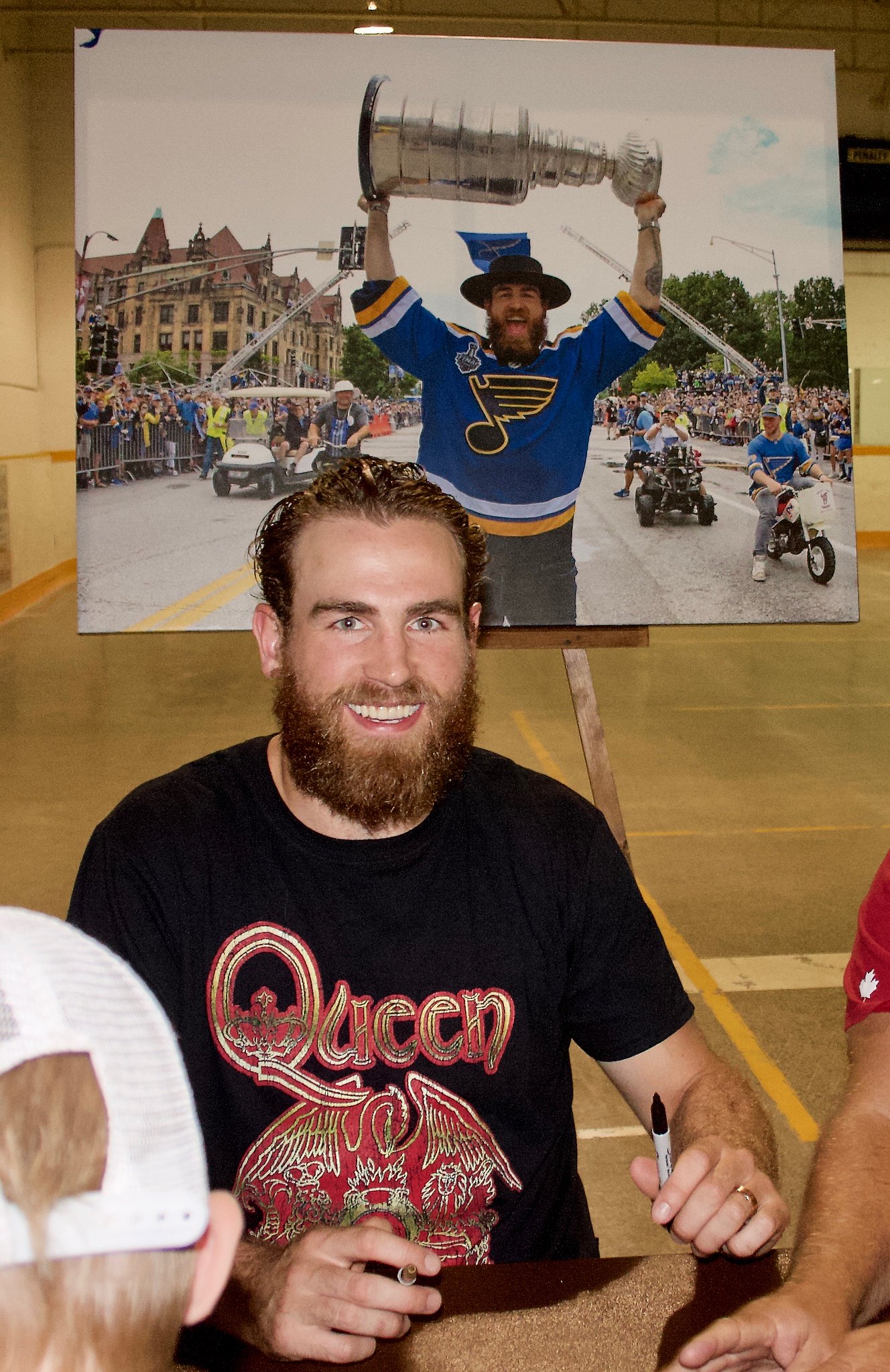In this photo, we see a white man in his late 20s to early 30s, possibly a professional hockey player, signing autographs. He is seated at a table with a tan granite-like surface and holds a black Sharpie in his right hand, which also sports a gold wedding band. He has short brown hair and a medium-length scraggly brown beard. The man is dressed in a black t-shirt featuring the "Queen" band logo in red and gold, along with an elaborate decal below it.

Behind him, displayed on an easel, is a poster board showing a photograph of the same man wearing a blue hockey jersey with black music symbols and white and yellow stripes. The image depicts him triumphantly holding the Stanley Cup above his head amidst a city street parade. The scene includes people crowding on either side of the road and some riding motorcycles or golf carts, with buildings and a line of trees in the background.

The setting for the autograph session appears to be a gymnasium, with other individuals partially visible around the man, including someone in a white hat and another with a red shirt sleeve. Although the children receiving the autographs are not fully visible, their presence is implied by the context.